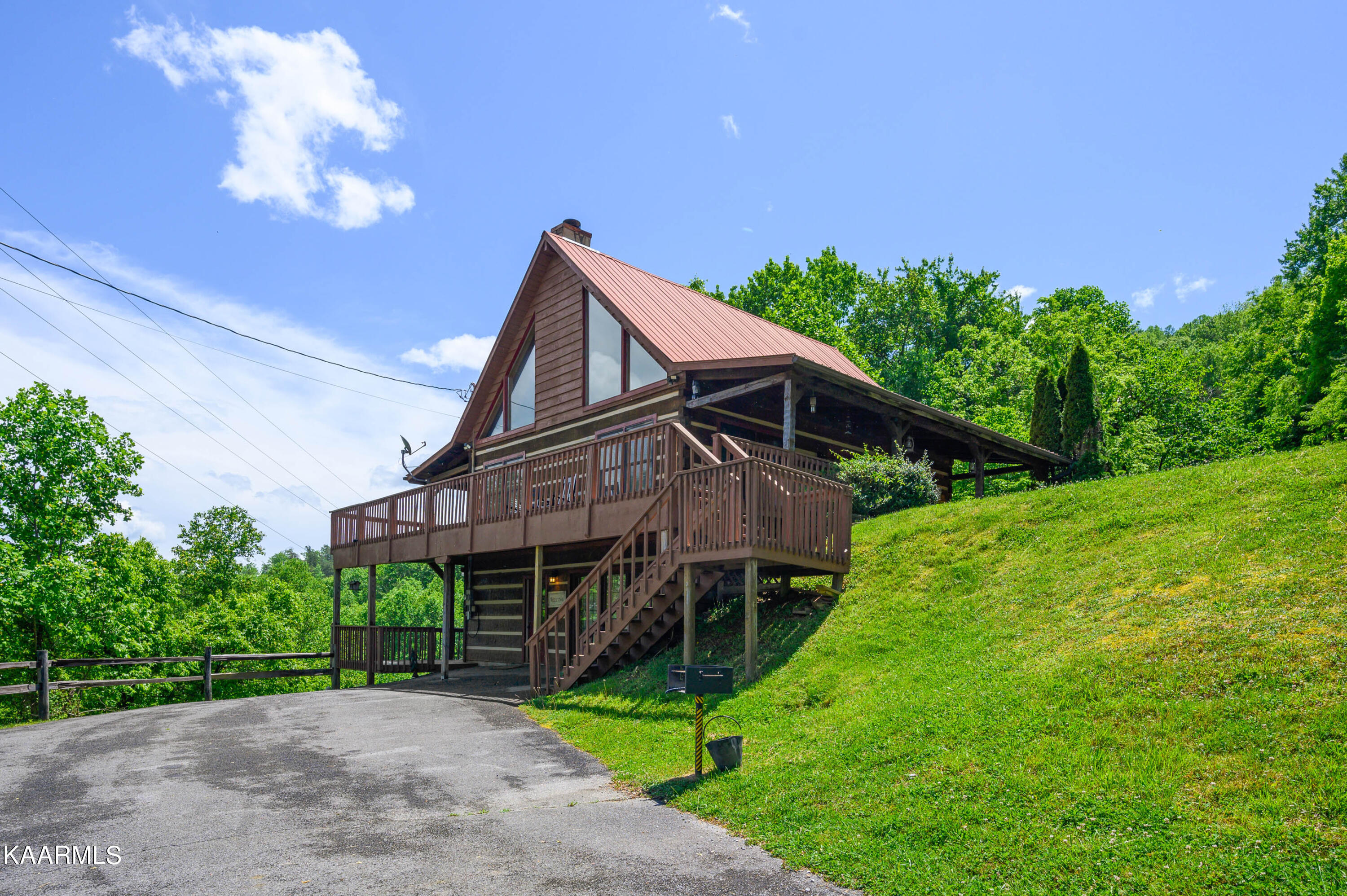The image depicts a picturesque outdoor scene featuring a western chalet-style house nestled into a green hillside. The sky above is a brilliant blue with sparse, wispy clouds. The background showcases a ridge densely packed with vibrant green trees, creating a serene natural backdrop.

The two-story house, prominently built into the slope of the hill, features a distinctive A-frame roof with triangular windows on the front. The top story boasts a wraparound porch, accessible by a set of stairs on the right side that rests against the grassy hillside. The house is predominantly light brown, with the lower level exhibiting a charming log cabin aesthetic composed of darker wooden planks. The upper balcony is supported by pillars rising from the lower level.

An asphalt driveway, grayish to dark gray and slightly sloped, leads up to the entrance of the house. Near the driveway, there is a black mailbox accompanied by a bucket. A wooden fence can be seen bordering the lower level. In the bottom left corner of the photo, the inscription "K-A-R-M-L-S" is visible.

Overall, the image captures the rustic beauty and unique architecture of the house, set against a lush, natural landscape bathed in daylight.